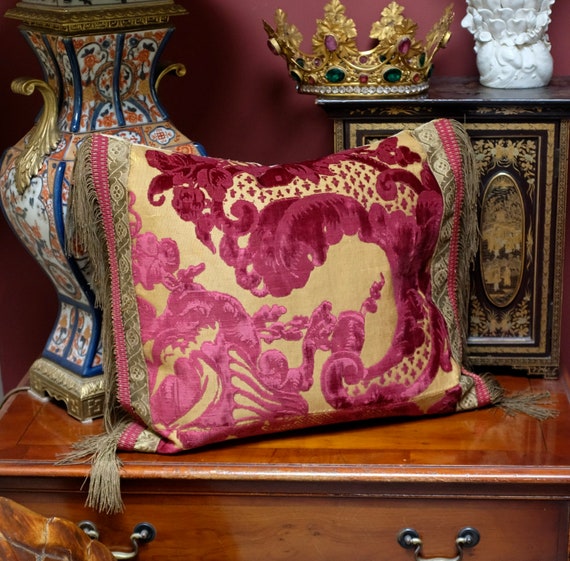The full-color vertically-oriented photograph, likely staged and taken indoors with artificial light, showcases a polished wooden cabinet adorned with two brass drawer handles at the bottom. On the cabinet's surface, a decorative pillow with tassels on its lower corners displays vibrant embroidery in shades of purple, red, yellow, and green, adding a burst of color. Behind the pillow stands an ornate vase reminiscent of Ming Dynasty designs, featuring a blue and white pattern with orange details, accompanied by gold accents at the base and sides. To the upper right, a small white figurine, possibly an angel, is perched atop a meticulously decorated wooden jewelry box, adorned with gold trimmings. Dominating the center of the upper section is an opulent golden crown, embellished with jewel-like decorations, lending an air of regality to the ensemble. The photo encapsulates a rich blend of textures and colors, creating a visually striking and detailed display.